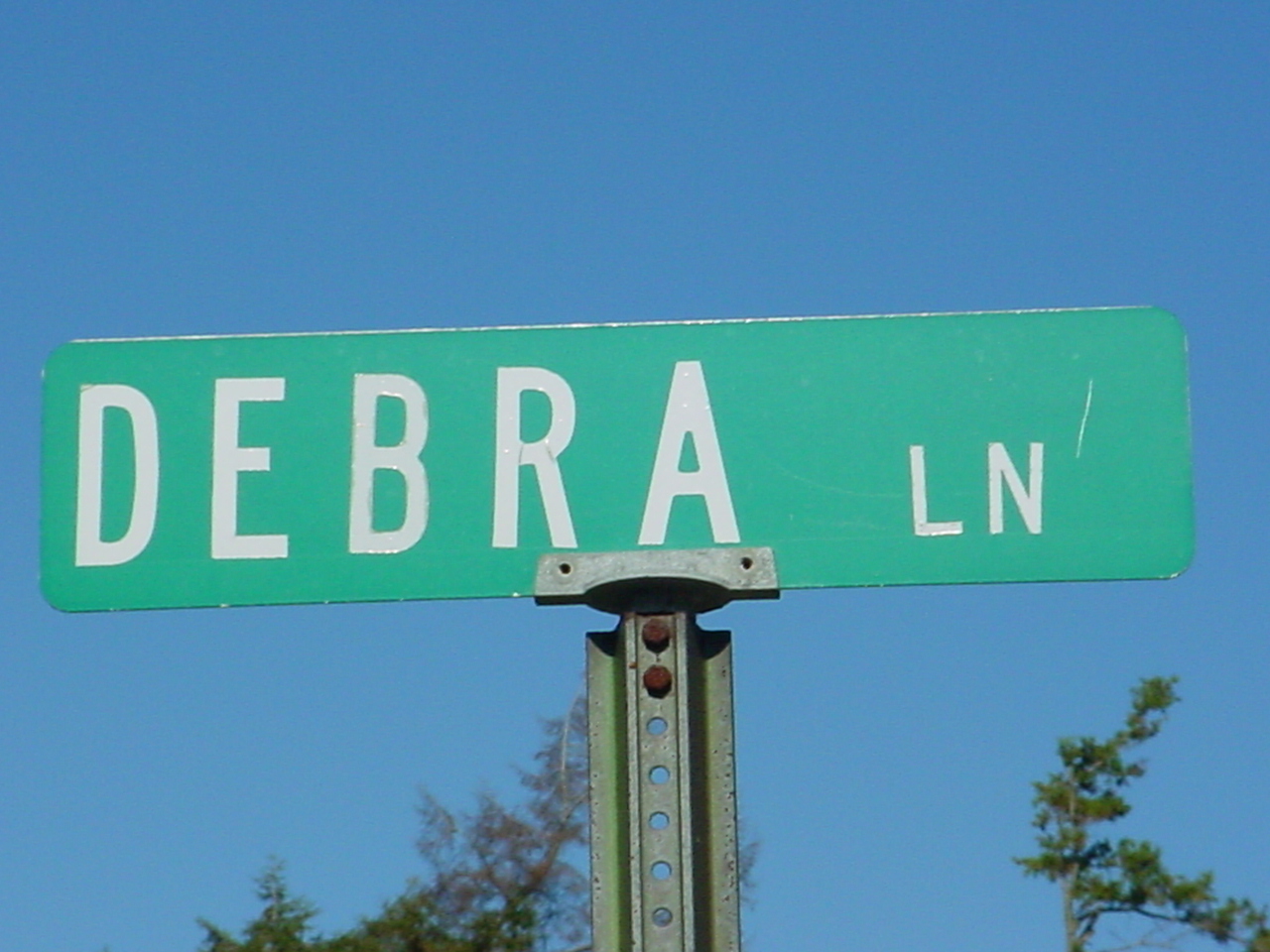A captivating outdoor photograph depicts a street sign captured from a ground-up perspective, showcasing the serene blue sky and the tips of lush, mature trees in the background. The sign is affixed to a sturdy metal post that extends from the ground up. The street sign, rectangular with gently rounded corners, stands prominently with its vibrant green hue. Its white reflective text clearly displays the name "Deborah Lane," offering a charming slice of everyday urban scenery.